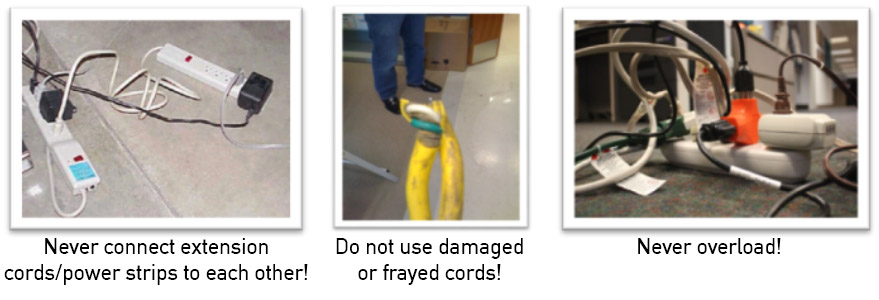This three-part image emphasizes safety with power cords and strips through clear examples and bold messages. The first image depicts a chaotic scene with two power strips and various cords overlapping and entangled, illustrating the caption "Never connect extension cords/power strips to each other." The second photo presents a damaged yellow cord with its green and white inner wires exposed, accompanied by a person's legs, underlining the message "Do not use damaged or frayed cords." The final picture features an overburdened extension cord with numerous devices stacked and plugged into it, reinforced by the exclamation "Never overload!" Each image serves as a cautionary illustration, warning against common electrical safety hazards.